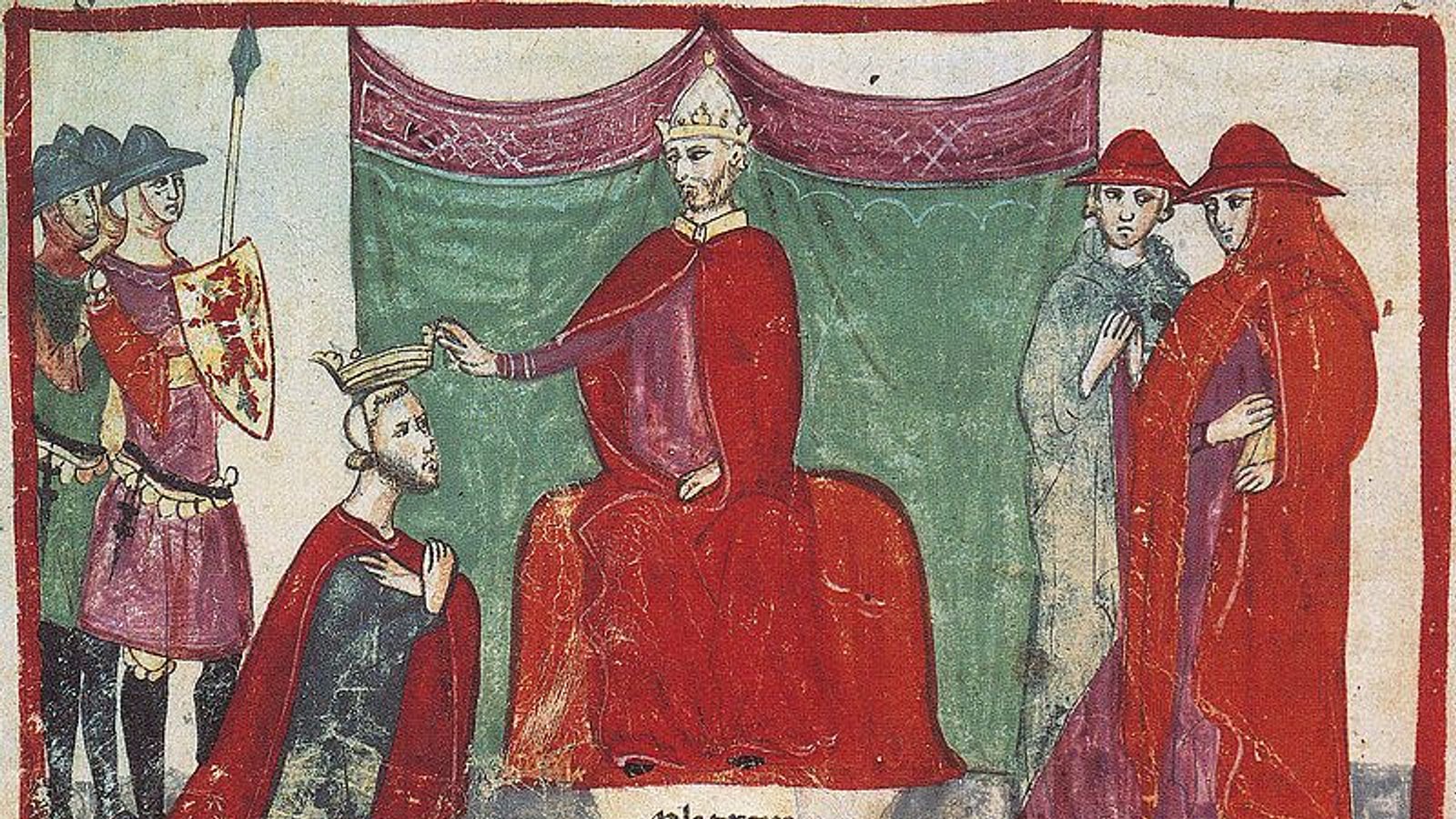The artwork is a medieval depiction, likely from the 12th century, showcasing a royal scene with a king bestowing a crown on a kneeling subject. Central to the image is a bearded man in elaborate red robes, seated on a throne-like red loveseat, his arm extended as he holds a crown above the head of a kneeling figure dressed in a red cape and a long black gown. The kneeling figure appears serene, with hands clasped near his chest.

Flanking this central action are six additional characters. To the left are two soldiers in distinctive attire: one in a pinkish-red outfit with long black boots, a black and gold belt, and a helmet, holding a shield adorned with a dragon and a sword, while the other, dressed in green, stands behind. On the right side, two figures in long robes—one in green with red accents and the other in red with a burgundy lining—observe the scene. They appear to be watching attentively, with one looking intently at the crowning and the other seeming concerned.

The scene is set against a green backdrop that resembles a tapestry, complemented by red detailing along the top. At the base of the throne-like seat is a plaque inscribed with the word "pla temp" in Gothic-like lettering, adding to the royal and historical atmosphere of the image. The style of the drawing is primitive and lacks realistic proportions and perspectives, characteristic of pre-Renaissance artwork.